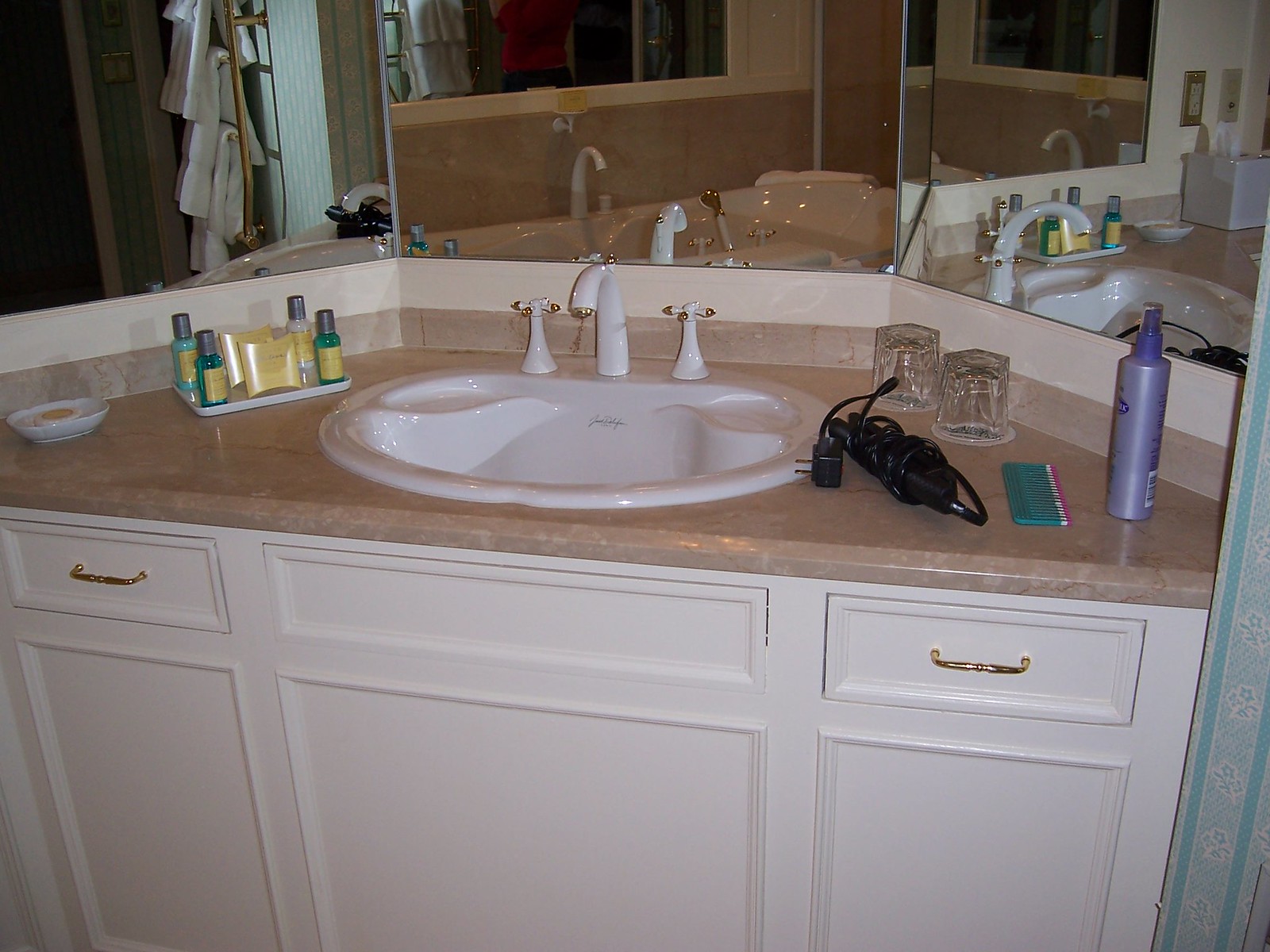This image showcases a luxurious bathroom area with an elegant white sink accented by gold trims and dual handles. The sink, which has a unique angled design, is centrally positioned and surrounded by three mirrors—flanking on the left and right, and one centered above it. On the sink counter, a black curling iron with its cord neatly wrapped around it is positioned, indicating readiness for use. To the left of the sink is a sophisticated soap display, which hints at a hotel setting. Adjacent to the display, reflected in the left mirror, we can observe a towel rack. 

On the right side of the sink, a vibrant purple shampoo bottle stands out on the brownish countertop. Nearby, two water glasses rest on paper coasters, oriented precisely for guest use. Additionally, a colorful detangler comb with hues of blue, white, and pink is placed near the water glasses. The sturdy sink vanity below includes two drawers, one on each side, each with a single, stylish gold handle, enhancing the coherent design theme.